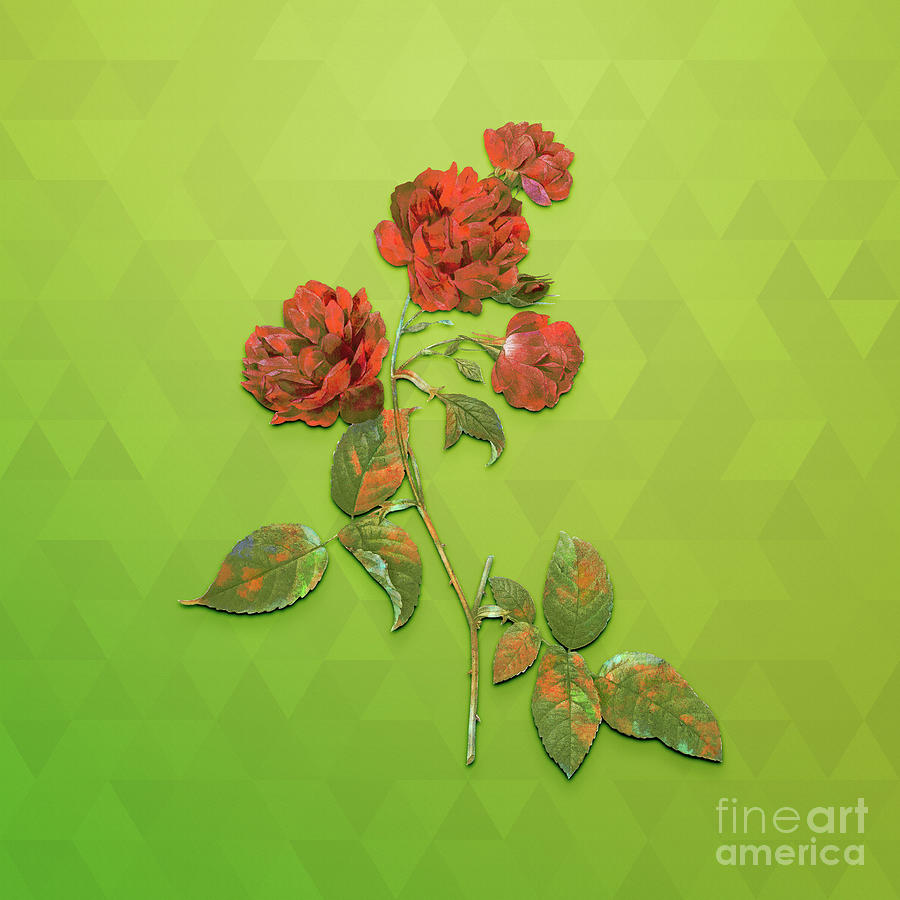This is a square image featuring a detailed digital art piece from Fine Art America, as noted by the watermark in the lower right corner. Dominating the composition is a rose stem with four red roses, each displaying nuanced shades of red to dark burgundy and accented with hints of green and brown on the petals. The stem centrally rises from the lower middle, curves gracefully to the left, then sweeps back to the right towards the top, showcasing several small offshoots. Surrounding the stem are clusters of leaves predominantly in forest green tinged with orange hues and sporadic blue spots, with a notable concentration on the lower right and middle left. The background enriches the artwork with a geometric pattern composed of various triangles and trapezoids, transitioning from a lighter olive green in the upper half to a slightly darker green in the lower left corner, adding depth and complexity to the visual narrative.